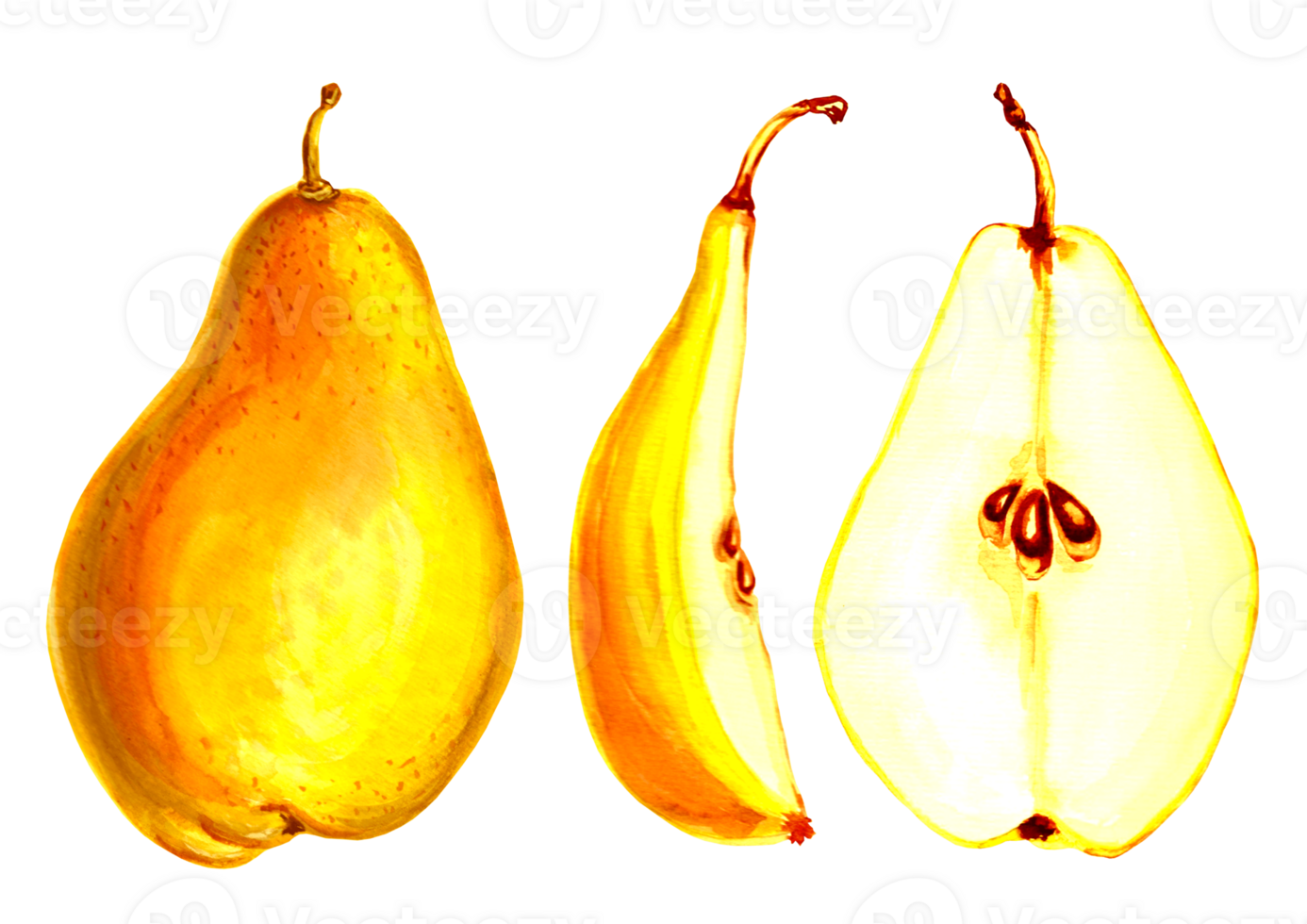The image appears to be a vibrant colored pencil drawing or colorful sketch featuring a pear depicted from various perspectives against a white background. On the left, a whole pear is shown upright, with its stem at the top and a skin characterized by various shades of yellow with slight freckling. The pear's rounded shape is more prominent on the left side. In the middle, the pear is cut into a slice, revealing the inner white and pale yellow flesh. This slice displays the outer yellow skin on the left, and on the right, the inner section with two small, teardrop-shaped brown seeds is visible. The rightmost image presents a direct view of the cut face of another pear slice, showing the smooth, pale flesh with three central seeds. The sleekness of the pear's interior contrasts with its slightly freckled exterior, all rendered in warm tones of yellow, brown, and orange.